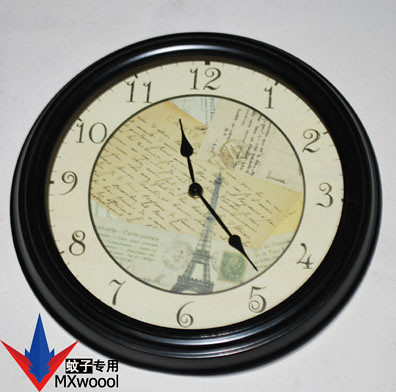The image showcases a circular, wall-mounted analog clock with a dark outer rim, which appears black or dark brown with a slight indentation. The clock's face is a cream or beige color, featuring a detailed design that includes an illustration of the Eiffel Tower prominently in the center. Surrounding the tower are numerous handwritten notes in yellow and white, layered atop each other, along with a small green stamp adjacent to the tower. The clock face also displays conventional numbers from 1 to 12 and has black hands; the shorter hand is just past 11, while the longer hand points slightly above 5. In the bottom left corner, there is a distinctive design consisting of a red-tipped, blue-bodied shape resembling an upside-down arrow. Additionally, the text "MXW000L" is visible, accompanied by some Asian characters. The clock is set against a light grey background.